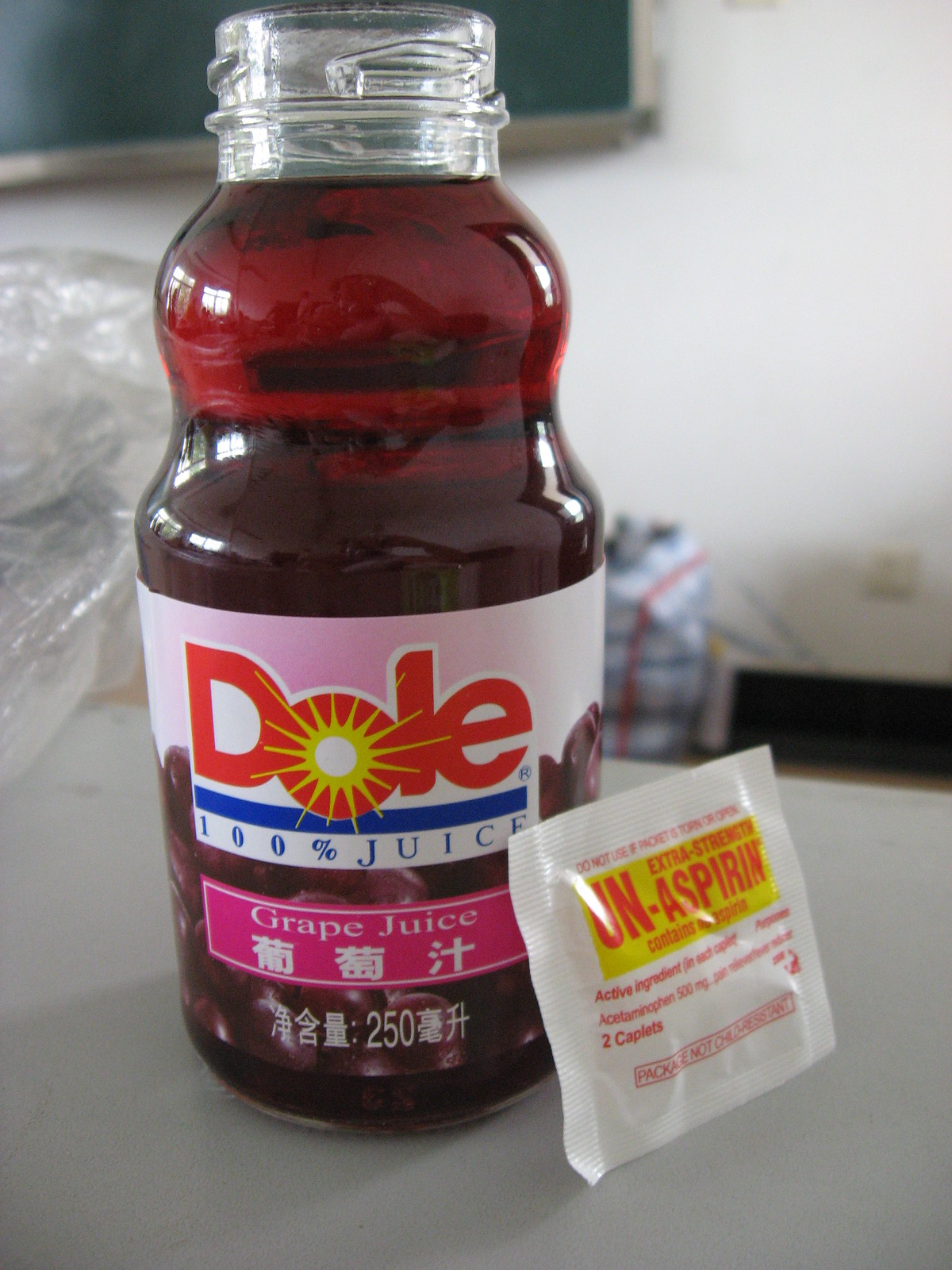The image depicts a Dole 100% grape juice bottle, which is full and has its cap removed. The bottle features both English text and Asian characters on its label, and the juice is a dark red color, akin to cherry red. The price on the label reads $2.50. Leaning against the bottle is a small white package of extra strength aspirin, which contains two caplets and has red lettering highlighted by a yellow box. The scene is set on a white table, likely in a classroom, as suggested by the green chalkboard in the background. Also visible are a plastic bag to the left of the bottle and another bag on the floor to the right.